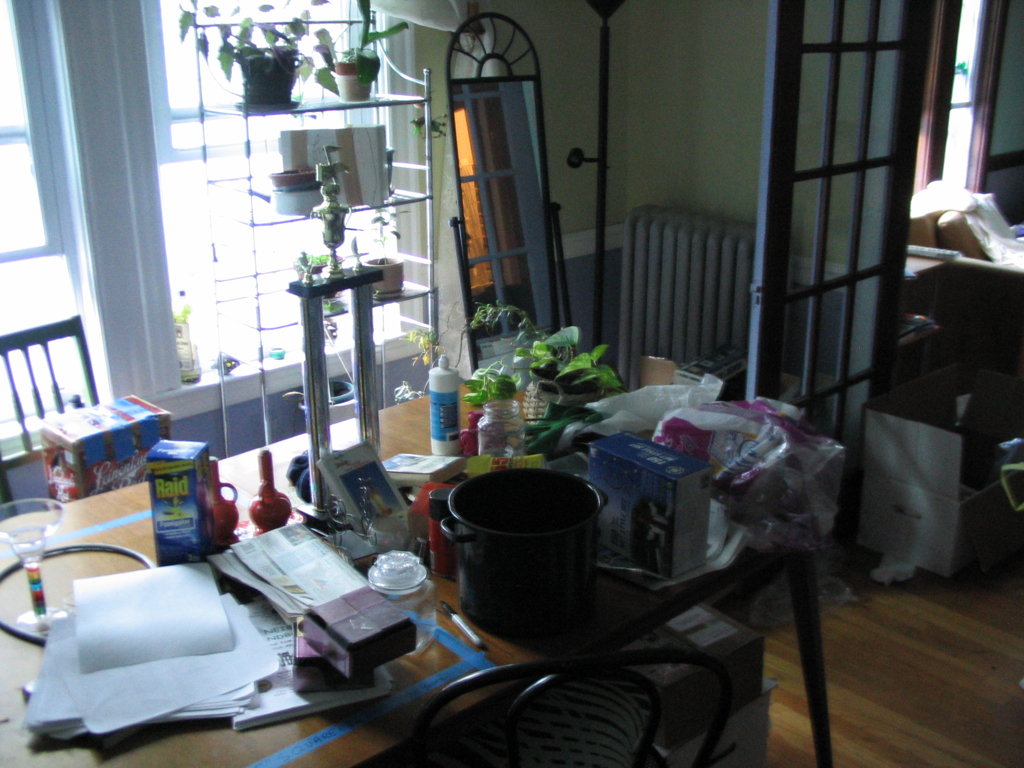This photograph captures the interior of a dining room in a house. Dominating the room is a large rectangular table situated in the center, accompanied by chairs on either side. The table is cluttered with various items, including a black pot, a tall trophy, a box of reed, a margarita glass, newspapers, and some plants, giving the scene a chaotic yet lived-in feel. 

On the left side of the image, near the top-left corner, there are two windows flooding the room with bright natural light. Positioned directly in front of the right window, there is a white plant shelf adorned with a few plants. Adjacent to this shelf on the right side stands a full-length mirror. Continuing further to the right, near the corner leading to the next room, there's a fixture that appears to be either a radiator or an air conditioning unit.

To the far right of the dining area, a glass door stands ajar, offering a glimpse into the adjoining room where a couch is visible, hinting at a cozy living space beyond.